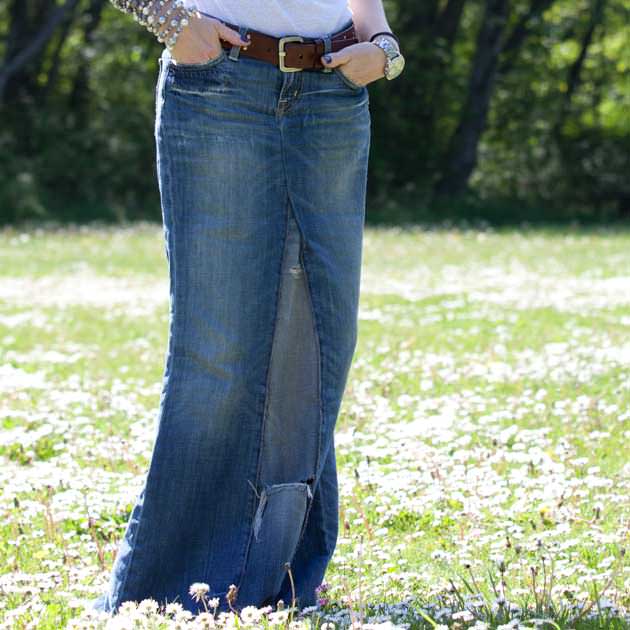The image depicts a young woman standing in an outdoor field of short green grass interspersed with white, puffy, dandelion-like plants and trees in the background. The perspective is from the waist down, showing her unique denim skirt, which appears to be creatively fashioned from a pair of jeans with the inseam cut out and additional denim sewn in to form the skirt. The skirt has a few ratty holes, suggesting a casual or DIY aesthetic. She's accessorized with a brown belt, multiple bracelets, a watch with a large face, and her hands are casually tucked into her pockets, displaying purple nail polish. Her outfit is complemented by a white top. The setting and the woman's attire give the impression that this is a candid shot, likely intended for social media rather than a professional product photo, showcasing her handmade fashion piece in a natural environment.